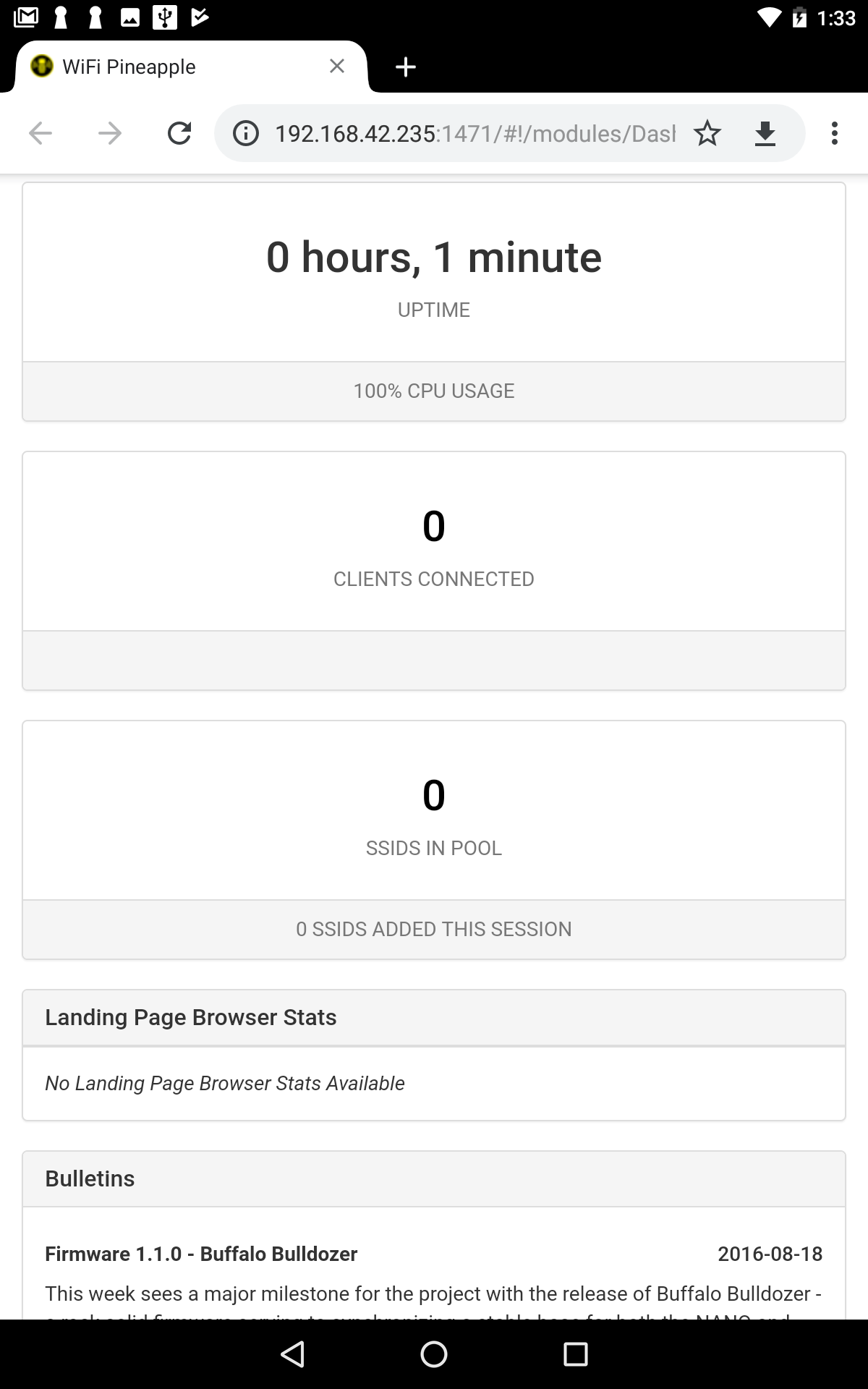The image is a vertical screenshot of a cell phone interface, taken from a device that is approximately 50% taller than it is wide. The screen has a primarily black background. 

In the top left corner, there are six icons; the first one is Gmail, and the others are not easily identifiable. In the upper right corner, the status indicators show full cellular signal strength, a mostly charged battery that appears to be charging, and the time, which is 1:33. 

Below the status bar is a single open tab labeled "Wi-Fi Pineapple." Adjacent to it on the right is a plus icon, indicating the option to open a new tab. 

The navigation bar below the tab includes standard icons for back, forward, refresh, a search bar displaying an IP address, and additional icons for favorites, downloads, and a menu represented by three vertical dots.

The main content of the screen is organized into several outlined gray boxes. The first box displays "0 hours, 1 minute" centered, under which it reads "uptime." Below this, it indicates "100% CPU usage."

The second box, positioned below the first, shows "0," with the smaller text below stating "clients connected."

The third box reads "0," followed by "SSIDs in pool."

Approximately 75% down the page, there is another box about half the height of the previous ones. This box is titled "landing page browser stats," with the text below stating "no landing page browser stats available."

Overall, the screen seems to be a monitoring interface for a network device, providing insights into usage and connectivity.